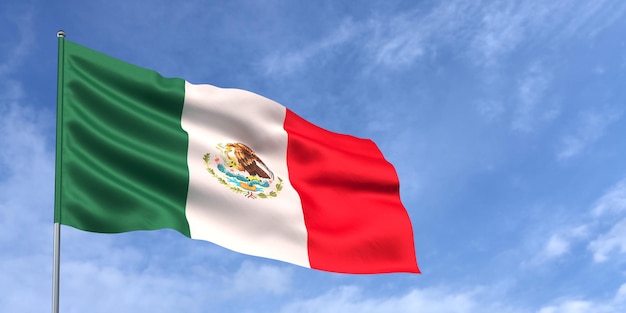The image depicts the Mexican flag, characterized by three vertical stripes in green, white, and red from left to right. The flag is blowing in the wind, evident from the soft ruffles and bends in the material. It is mounted on a tall silver flagpole, extending up into a bright blue sky adorned with white puffy clouds. The photo is taken from a ground-level perspective, angled upwards towards the flag. In the center of the white stripe, there is an intricate emblem featuring a brown eagle perched on a green cactus, which is surrounded by water. The emblem underscores the cultural and national symbolism of the flag.